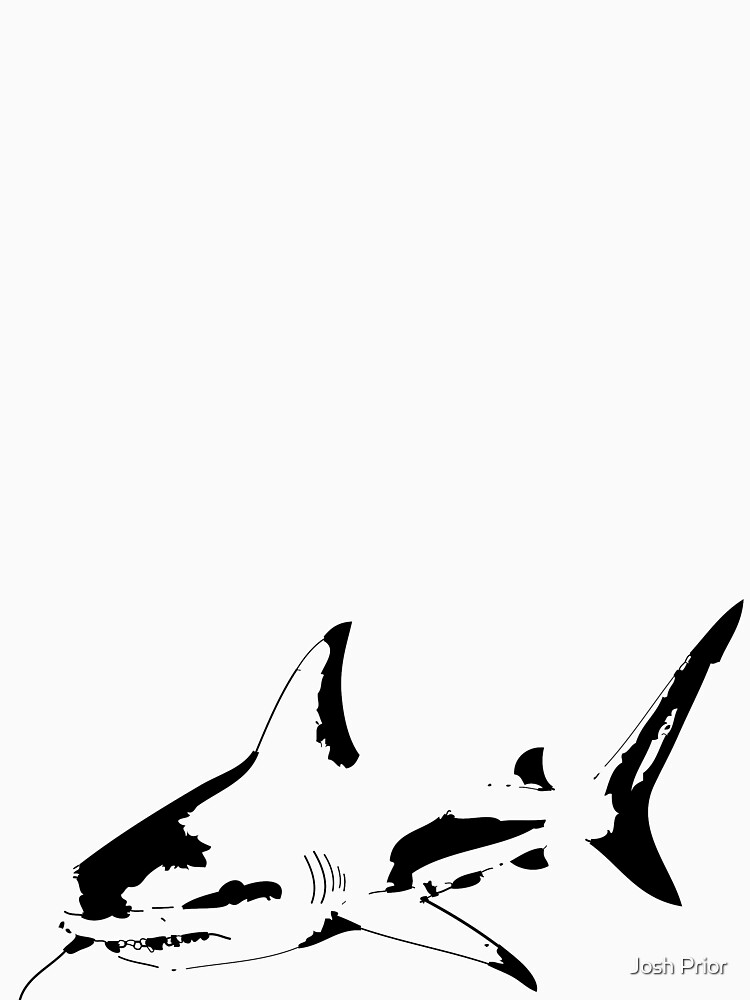This image depicts a striking, artistic rendering of a shark set against a clean, white background. The shark, positioned at the very bottom of this large, vertically oriented image, features an intricate blend of line drawing and abstract black blobs. These blobs, strategically placed on parts of the shark such as its dorsal fin, pectoral fins, tail fin, and head, prompt the viewer to fill in the details using their imagination, utilizing the negative space to complete the form. The shark’s body is primarily white, contrasted sharply by black spots and lines, including detailed black markings on its fins, tail, and around its eye. The image evokes a sense of minimalist design, with ample empty white space above the shark, making it appear almost like a piece of modern art or a potential wallpaper for a phone. In the bottom right corner, the name "Josh Pryor," presumably the artist, is written discreetly. The overall color palette is monochromatic, featuring shades of gray, white, and black, adding to the image's stark and captivating aesthetic.